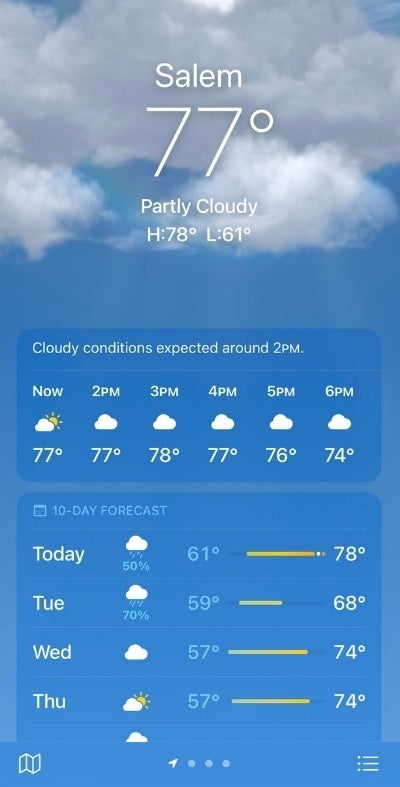Screenshot of a weather forecast from Weather.com with a serene baby blue backdrop. At the top, fluffy white clouds decorate the background. The main part of the screen features a detailed weather summary for Salem, Texas, displaying a current temperature of 77°F, with "Partly Cloudy" conditions and a high of 78°F and a low of 61°F. Below, there's a darker blue box warning of cloudy conditions expected by around 2 p.m., with an hourly forecast spanning from "Now" through 6 p.m. The "Now" segment shows a cloud icon with a hint of sun, followed by consistent cloud icons for the subsequent hours along with temperatures: 77°F, 77°F, 78°F, 77°F, 76°F, and 74°F.

A separate gray box labeled "10-day forecast" presents a concise overview:
- Today: 50% chance of rain, highs of 78°F and lows of 61°F
- Tuesday: 70% chance of rain, highs of 68°F and lows of 59°F
- Wednesday: Cloudy, highs of 74°F and lows of 57°F
- Thursday: Cloudy with partial sunshine, highs of 74°F and lows of 57°F

At the bottom of the screenshot, there's a map on the left, a GPS icon in the center, and three dots with lines on the right, completing the interface.